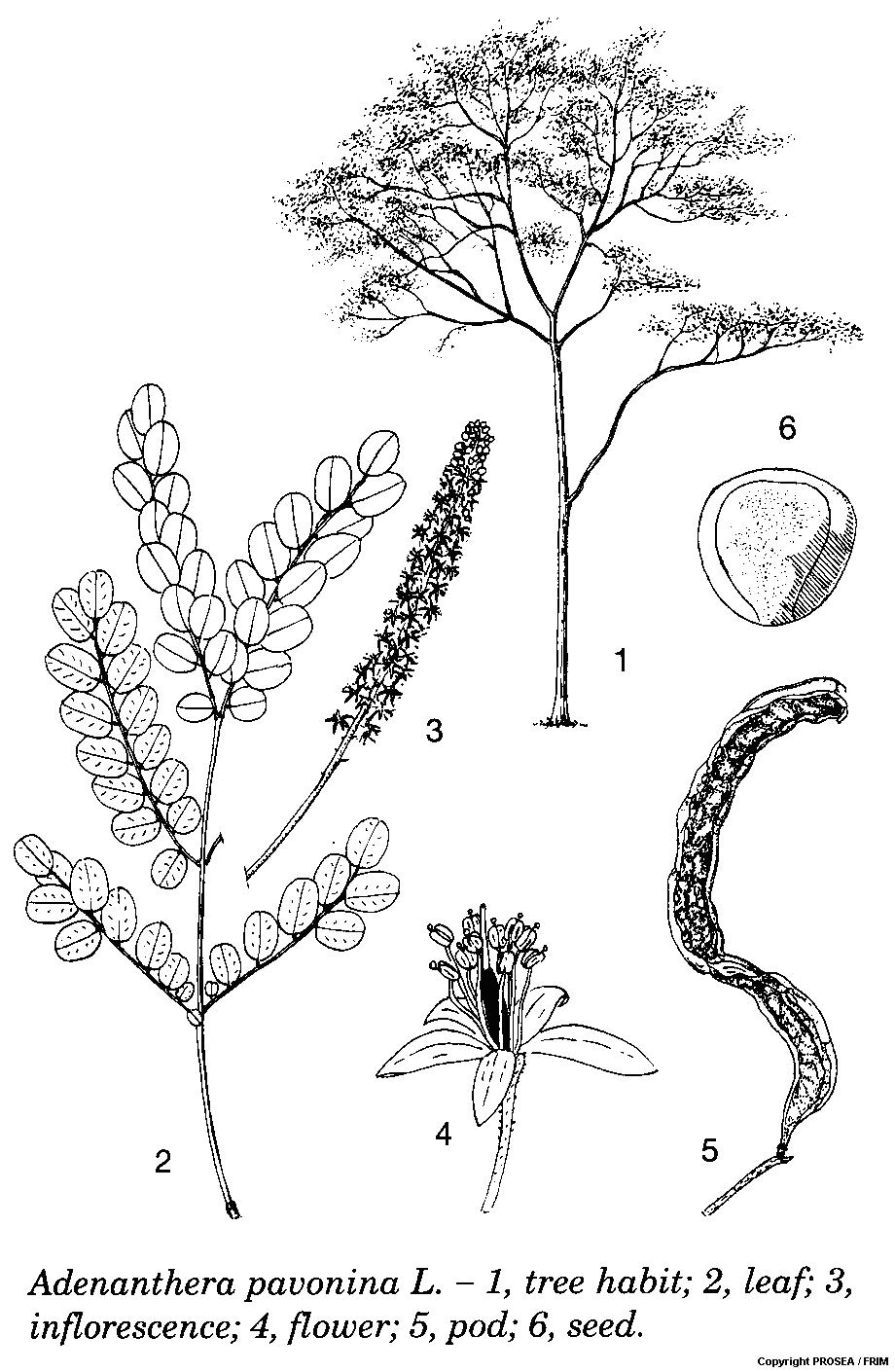This detailed illustration, likely sourced from a science textbook, depicts various parts of the tree Adanthera pavonina. The hand-drawn, black and white diagram is divided into six labeled sections. Number one, "Tree Habit," showcases the overall structure of the tree, featuring sparsely spaced branches with a concentration of small, short, oval leaves at the top. Number two, "Leaf," highlights these leaves in detail, displaying a central line and tiny dots on the surface. Number three, "Inflorescence," illustrates a densely clustered branch with small, sharp, pointy leaves. Number four, "Flower," presents the flower in full bloom with open petals, a tall pistil, and slender stems topped with buds. Number five, "Pod," resembles a string bean, elongated with internal structures reminiscent of beans. Finally, number six, "Seed," is depicted as a round object with speckles, complete with an internal circle. The accompanying key at the bottom clearly labels and describes each part of the Adanthera pavonina tree.